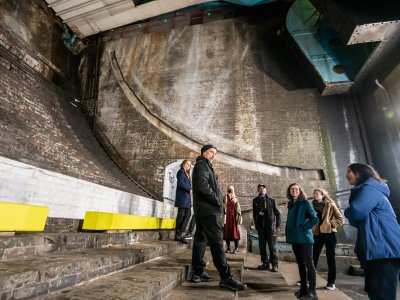In the image, a group of eight people is seen standing on concrete steps within a large warehouse-like structure, characterized by its high ceiling and expansive headroom. The environment appears dank and slightly humid, with dirty walls that suggest a lack of regular maintenance. The central point of the image showcases these individuals, all bundled in jackets and pants, indicating cold weather. Some of the people are wearing IDs, enhancing the sense of an organized visit, perhaps a tour or an inspection.

The setting is quite complex, featuring various structural elements: yellow rectangular horizontal beams, white barriers, and seats that create a confusing mix between an auditorium and industrial space. Behind the group, there are yellow bench-like chairs in front of white seating, adding to the peculiar ambiance. The background reveals large brown and stone walls with a distinct curve that almost seamlessly merges into other elements like high-tension wires. A blue-toned ceiling gives an additional layer of intrigue to the space. 

Each person appears distinct in their attire – noticeably, there's a person in a blue coat on the far right, another in a green coat centrally positioned, one in a brown coat, someone in a black coat and pants with a hat, a person in a leather coat with a cloth cap, and another in blue and red outerwear. Their body language suggests a casual gathering, with some individuals having their hands in their pockets or arms folded, implying they are slightly uncomfortable, possibly due to the cold.